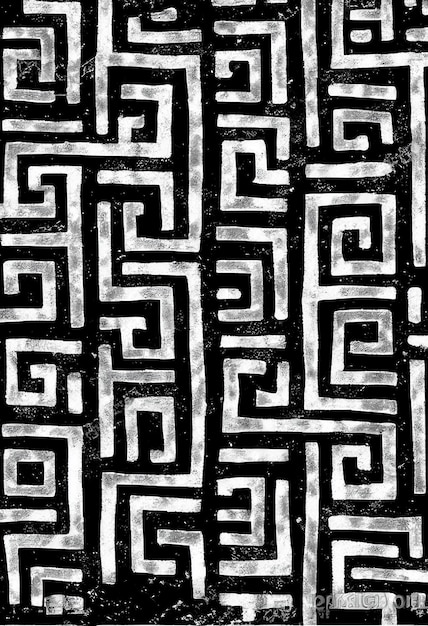The image features a rectangular piece of artwork, with its length twice its height. It showcases an intricate pattern of thick black and white lines set against a black background. These lines intersect at right angles, creating a maze-like, non-repeating and deconstructed array of shapes that include backward L's, shapes resembling the number nine, and barbell-like forms. The lines are detailed with various shades of gray and white spots, giving the artwork a faded, textured look. Despite a watermark present in the bottom right corner, it remains unreadable due to the low resolution of the image and its camouflage within the complex pattern.